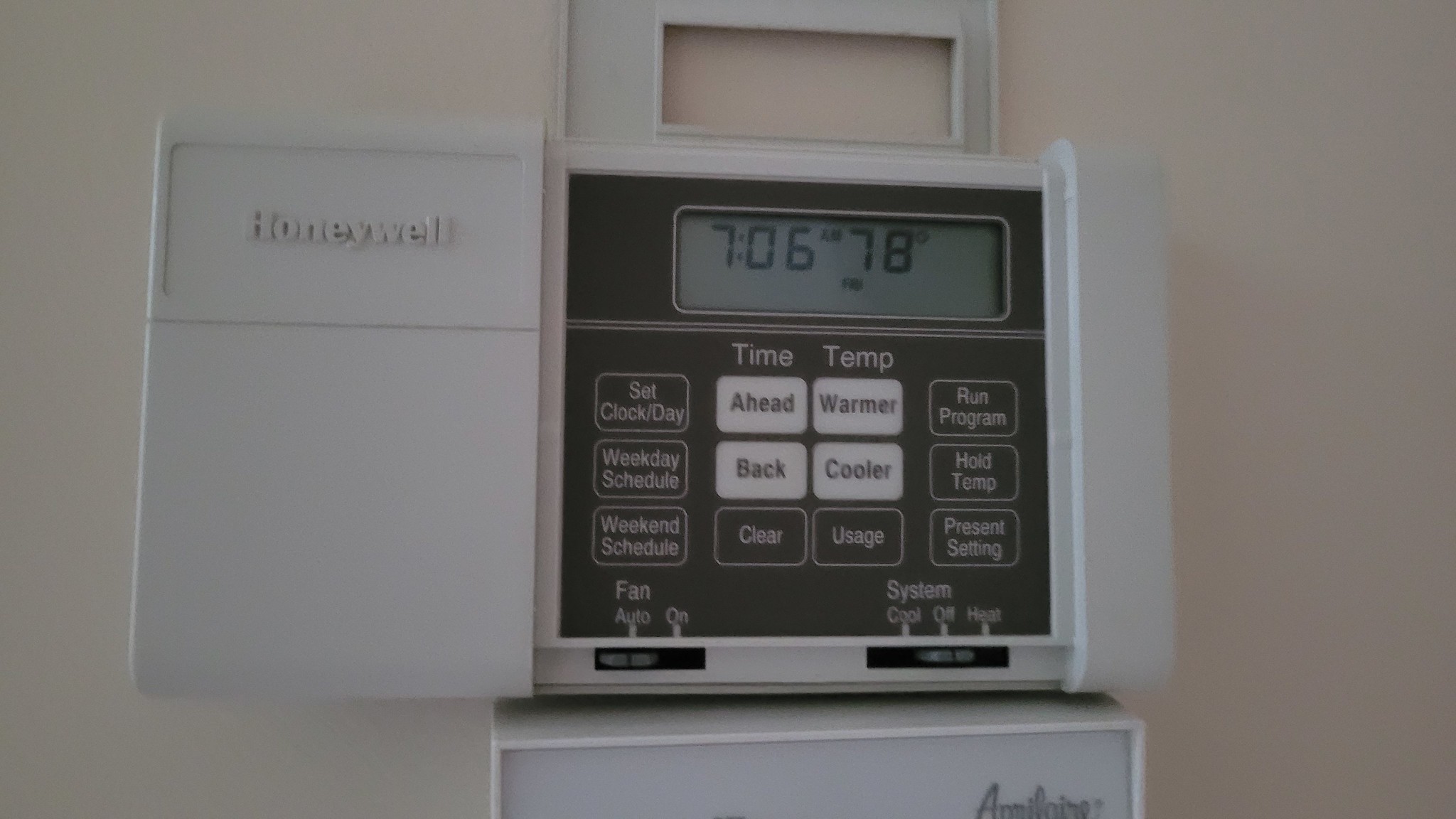Close-up of a Honeywell thermostat mounted on an eggshell-colored wall. The white plastic panel is slid to the left, revealing the display and control buttons. The display indicates that the current time is 7:06 a.m. and the temperature is 78°F. Below the display, there are several clearly labeled buttons. They include options for adjusting the time (ahead, back, and clear) and the temperature (warmer, cooler, and usage check). To the left, additional buttons provide scheduling options, such as setting the clock and day, configuring a weekday schedule, or a weekend schedule. On the right, there are program controls to run the program, hold the temperature, and present settings. The fan can be set to auto or on, while the system can be switched between cool, heat, or off. Beneath the thermostat, there is another white plastic box featuring a brand name in silver print, "Amilair."